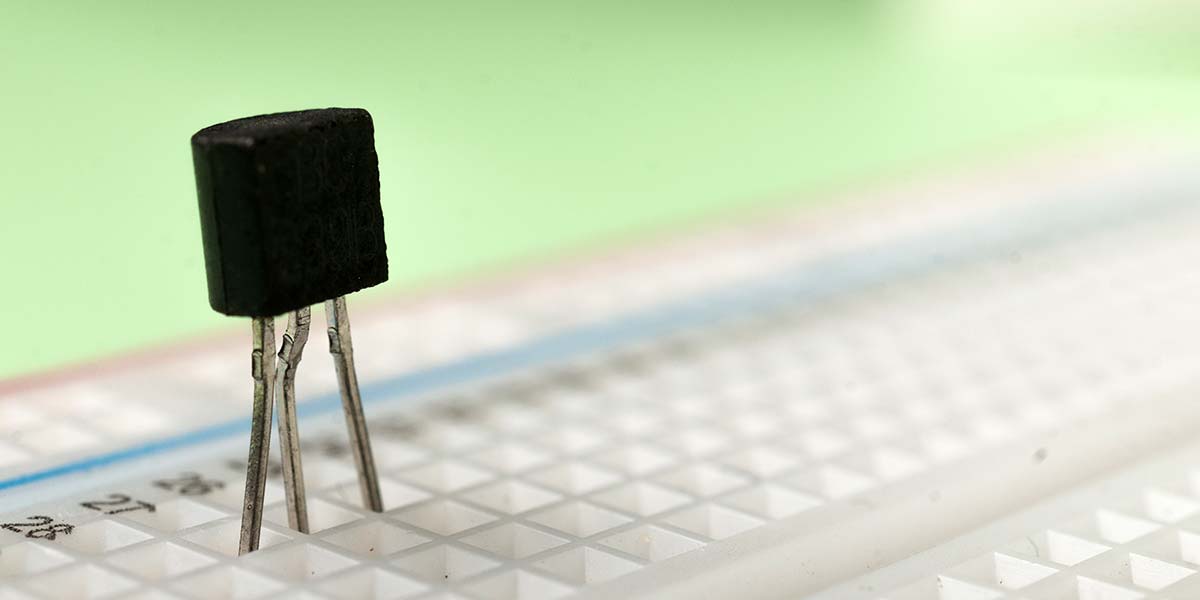This image depicts a detailed close-up of a white, plastic grid structure composed of evenly spaced, small square compartments. A column along one side is sequentially numbered with black digits, such as 28, 27, 26, and 25, running downward. Within the grid, positioned precisely between the numbers 25, 26, and 27, is a small black toggle switch. This switch features a black button with three silver metal legs extending from it, anchored into the corresponding numbered squares. Additionally, the upper half of the image is characterized by a blur of light green color in a diagonal orientation, adding contrast to the structured grid below. This arrangement suggests the presence of an electronic component, possibly used in soldering practice or as part of a training kit for assembling hardware.